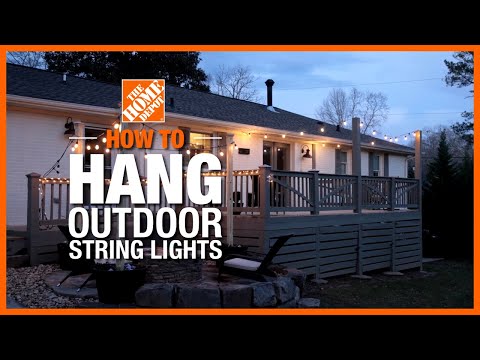The image is a late advertisement for Home Depot, featuring a picturesque single-story house typical of an American neighborhood. The home has white siding, a blue roof studded with vents and poles, and a wooden deck adorned with small, orange string lights that illuminate both the deck and one side of the house. A stone fire pit is also visible, with trees forming a serene backdrop. The scene is captured at twilight, with the sky transitioning from blue to a darker hue.

The photograph is framed with an orange border, reminiscent of the Home Depot’s signature color. Overlaying the image, there is a prominent Home Depot logo. In the center, large, bold white text states, "Hang Outdoor String Lights," with "Hang" being the largest word. Below it, in smaller orange letters, it says "How to." The overall composition suggests this is not just an advertisement but part of an instructional series, likely a leaflet or manual from the DIY store, aimed at guiding customers on how to hang outdoor string lights effectively. The deck lights add a festive, inviting glow to the serene evening scene.